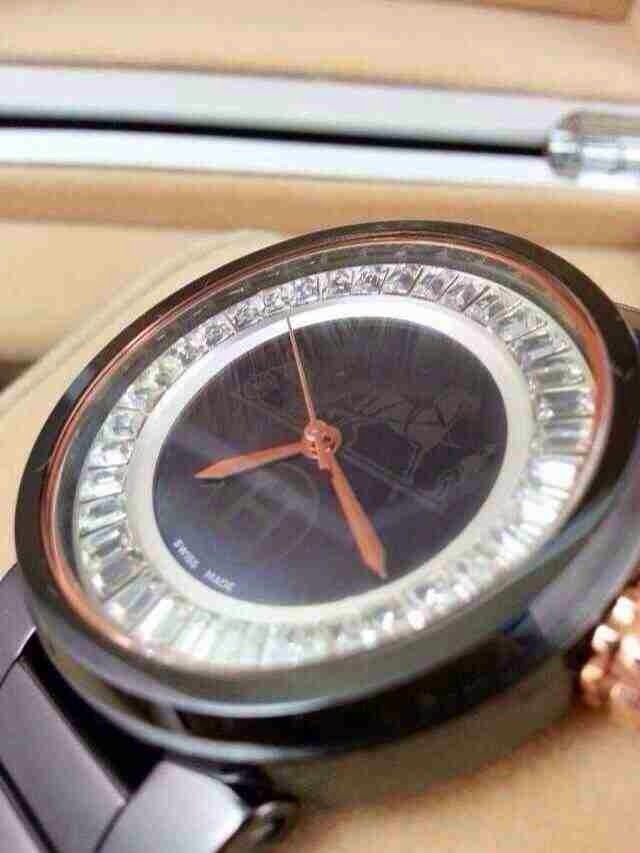The image features an extreme close-up of a high-caliber wristwatch. Despite the very poor quality resulting in visible noise, pixelation, and distortion, distinct details can still be discerned. The circumference of the watch face is encrusted with small diamonds, adding a touch of luxury to its appearance. The watch face, devoid of numbers, prominently displays three hands - hour, minute, and second - indicating a time of approximately 7:20. At the 6 o'clock position, amidst the dark black face, the blurred yet readable white text reads "Swiss-made," attesting to the watch's quality and origin. The wristwatch is accompanied by a dark grey gunmetal-colored strap, with the linkages visible at the bottom of the image. The backdrop suggests a soft, velvety felt material, likely the interior of the watch's case, hinting at the luxurious packaging. The watch appears to be resting on a soft cushion, partially visible, within a beige-colored case, providing a fitting display for this refined timepiece.